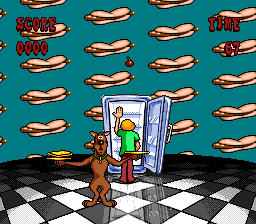This image depicts a scene from a Scooby-Doo and Shaggy video game, presented in a small square format. The background features a blue backdrop adorned with vertical rows of hot dogs stretching across the entire image. Positioned centrally, Shaggy is seen from behind as he peers into an open refrigerator, its door swung open to the right. Shaggy stands directly in front of the refrigerator, engrossed in its contents. In the foreground on the left, Scooby-Doo is holding two plates of food, one in each hand—his left hand elevated slightly higher than his right. The floor beneath them is designed in a classic black-and-white checkered pattern, adding a retro touch to the scene. At the top left corner of the image, game interface elements are displayed: the word "Score" in red, followed by "000", and "Time" also in red, showing "67" seconds remaining.